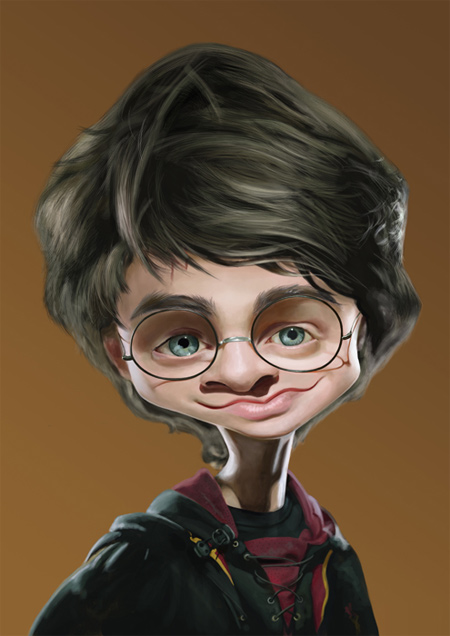This image is a detailed computer graphic drawing of a young boy whose appearance resembles Harry Potter, though his face is notably distorted. He has messy, somewhat long black hair that partially covers his forehead and may obscure a hint of a scar. His unusually large, green eyes peer through round glasses similar to those worn by Harry Potter. The boy's mouth and chin are notably constricted, giving his face a scrunched-up look, while his neck appears unusually thin. He wears a burgundy hoodie under a black jacket, which may have hints of yellow lines, and a possibly dark purple or black t-shirt underneath. The background of the image is a plain, uniform brown, and the composition is drawn in portrait orientation.